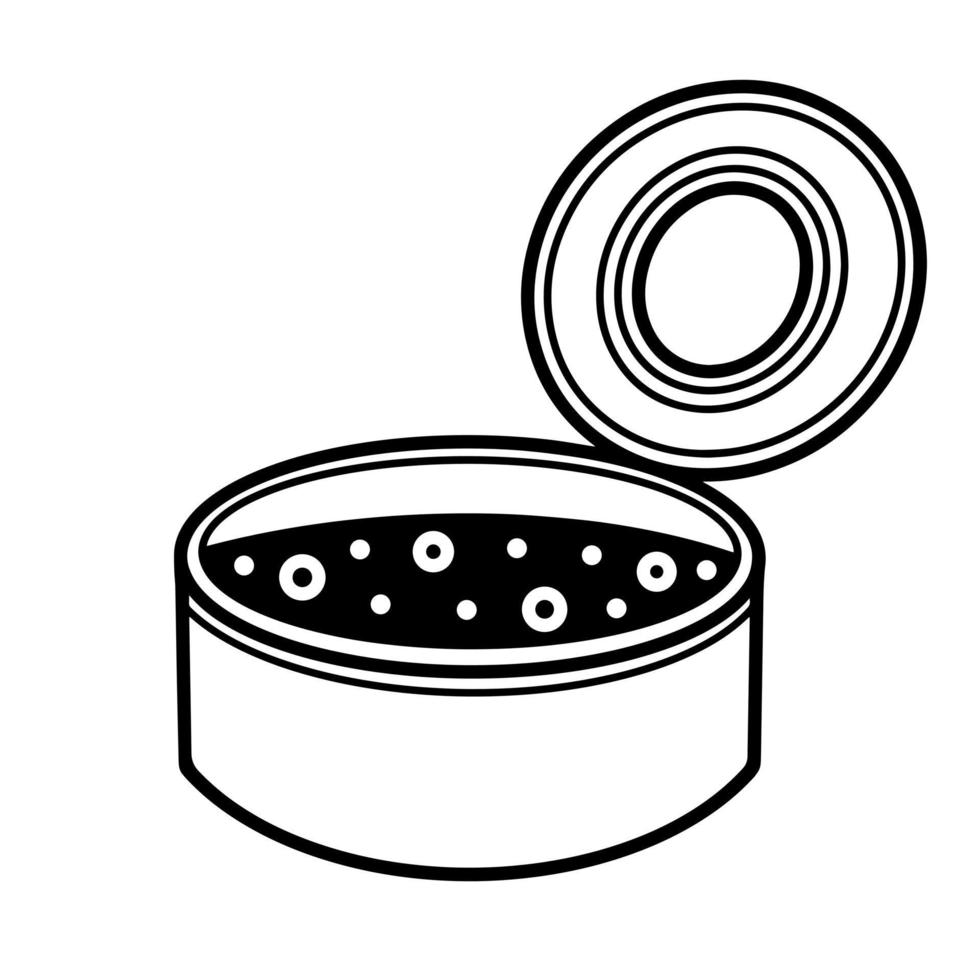The image is a detailed black-and-white cartoon drawing of a tin can, roughly the size and shape of a tuna can, making it shallow, short, and round. The tin's lid has been partially opened with a can opener and is flipped up to the right. The interior of the can appears shaded in black with numerous white circles, possibly reminiscent of fish eyes, to indicate texture. Similarly, the lid itself features concentric circles for added texture. This clipart-style image is set against a plain white background, highlighting its simple yet detailed design.